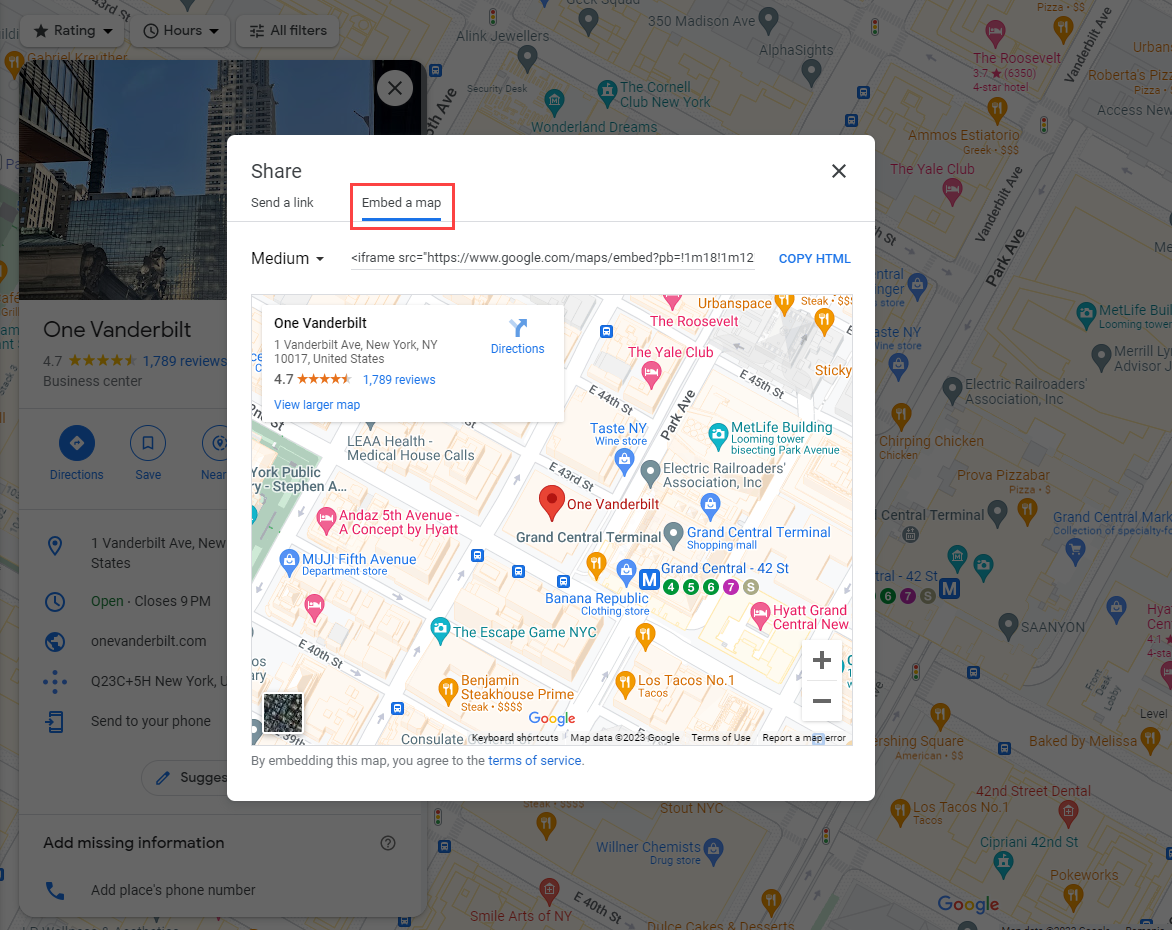The image appears to be a detailed screenshot of a Google Maps page for One Vanderbilt Avenue in New York City. The image features a gray, out-of-focus border, with the top section displaying options like "Rating," "Hours," and "All Filters."

In the main section, it showcases One Vanderbilt with a 4.7-star rating, based on 1,078 reviews. It is identified as a business center, with a blue circular button labeled "Directions." The address is provided as One Vanderbilt Avenue, New York, NY, 10017, accompanied by a link to its official website, onevanderbilt.com.

Additional options are given for sending the information to your phone, adding missing information, and adding places. The phone number and other associations, such as the Electric Railroad Association at 463, and mentions of places like "Tacos Number One" and "Wonder Chemist," are also included.

The bottom section of the image features a square with options to share or send a link, and it is bordered in red. There's an embedded map with an iframe source URL pointing to Google Maps. The map highlights One Vanderbilt Avenue, Grand Central Terminal, the MetLife Building, and other nearby landmarks, like "Benjamins," "Steakhouse Prime," and "New York City."